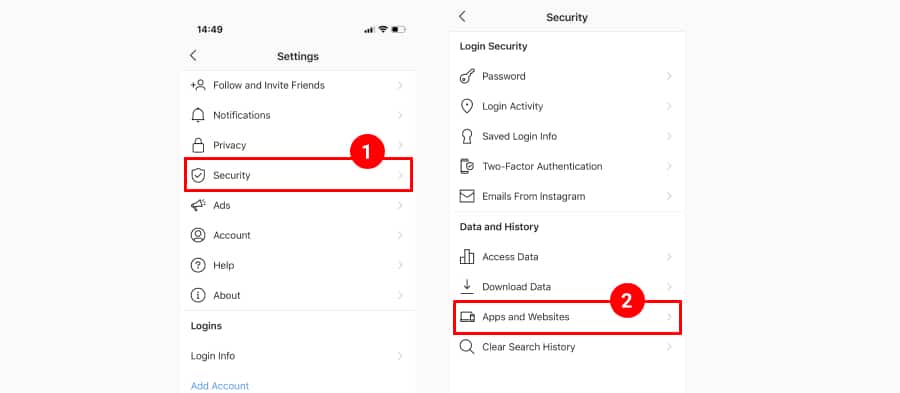This is a detailed caption for an instructional image showing how to navigate the security settings on a cell phone. The screenshot is divided into two distinct sections. 

On the left side, the image displays the "Settings" menu, highlighting various options including "Follow and Invite Friends," "Notifications," "Privacy," "Security," "Ads," "Account," "Help," "About," "Logins," "Login Info," and "Ad Account." The "Security" option is emphasized with a red box and a red circle containing the number "1." 

On the right side, the image focuses on the "Security" submenu where users can find options like "Login Security," "Password," "Login Activity," "Saved Login Info," "Two-Factor Authentication," and "Emails from Instagram." Below these, there is another section labeled "Data and History" which includes options such as "Access Data," "Download Data," "Apps and Websites," and "Clear Search History." The "Apps and Websites" option is marked with a red box and a red circle containing the number "2." 

The key purpose of the image is to guide users through accessing the "Apps and Websites" selection within the security settings of their cell phone, using bright red markers for clear visual emphasis.